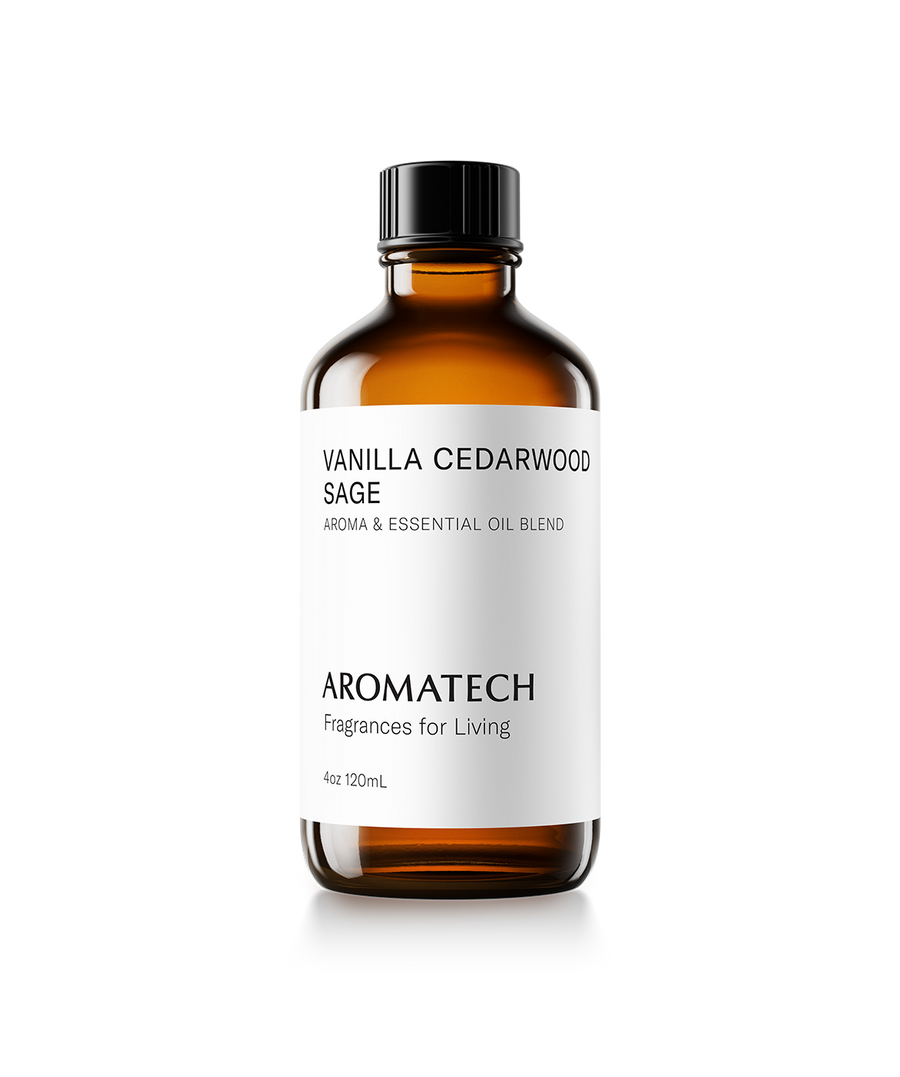The image features a detailed photograph of an essential oil blend from Aromatech. The label at the top of the bottle prominently displays the words "Vanilla, Cedarwood, Sage, Aroma, Essential Oil Blends" in black text on a white background. Towards the bottom of this label, the brand name "Aromatech" is printed in large, bold, black capital letters. Below the brand name, the tagline "Fragrances for Living" is written in smaller, elegant letters. The label also indicates the volume of the bottle, which is 4 ounces (120 milliliters).

The bottle itself is made of brown glass and appears completely filled with the essential oil blend. The cap sealing the bottle is a very dark black, providing a contrasting look against the brown glass. This product is likely intended for use in an oil diffuser or for home fragrance purposes. The scent combination—vanilla, cedarwood, and sage—suggests a soothing and aromatic experience. The presentation and labeling indicate that this is a commercial product aimed at enhancing the ambiance of living spaces.